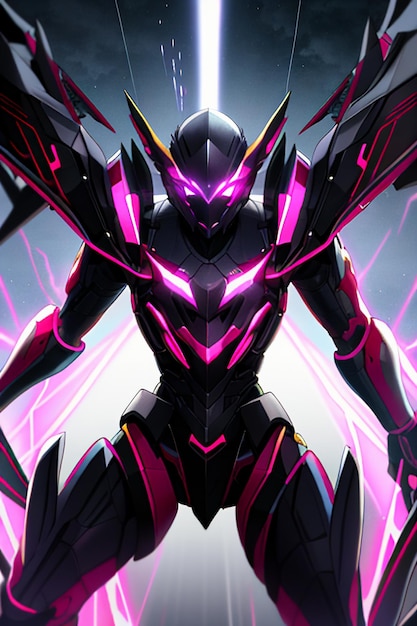This captivating fantasy digital image showcases an anime-style robot or alien character, entirely encased in a sleek, black battle suit adorned with glowing purple neon accents. The character's imposing helmet features distinctive long, upward-pointing wings that frame a pair of striking, glowing purple eyes. Complementing the helmet, the shoulders of the suit are equipped with equally large, wing-like protrusions, also extending upward. The armor is further embellished with glowing purple highlights, especially noticeable on the chest piece and various parts of the suit. Additional elements of the design include long, sharp spikes extending from the thigh areas of the armor. The dynamic background features vibrant purple laser-like energy beams that add depth and intensity to the image, creating a mesmerizing sci-fi atmosphere.